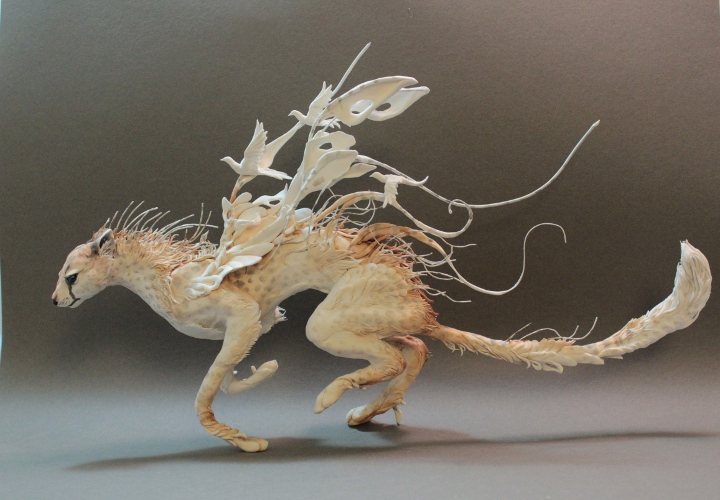This is an image of a fantasy interpretation of a cheetah with elongated and exaggerated features, making it appear somewhat akin to a weasel or otter. The cheetah's pale yellow body is adorned with very light gray and tan spots, appearing darker toward its hindquarters. Its limbs, particularly the front ones, bend unnaturally, emphasizing its motion as it runs from right to left in a profile shot. Accompanying its lithe form is an unusually long tail that flares out to a poofier end. The cheetah is depicted with striking black eyes and a black nose, with wings emerging majestically from its shoulder blades. Enhancing its mystical appearance, white doves are in flight above these wings. The cheetah’s body also transitions from shorter hair at the neck to longer hair toward the tail. The background of the image is a dark grayish-brown, creating a stark contrast that highlights the ethereal and otherworldly nature of the running cheetah, its wings, and the flock of accompanying birds.